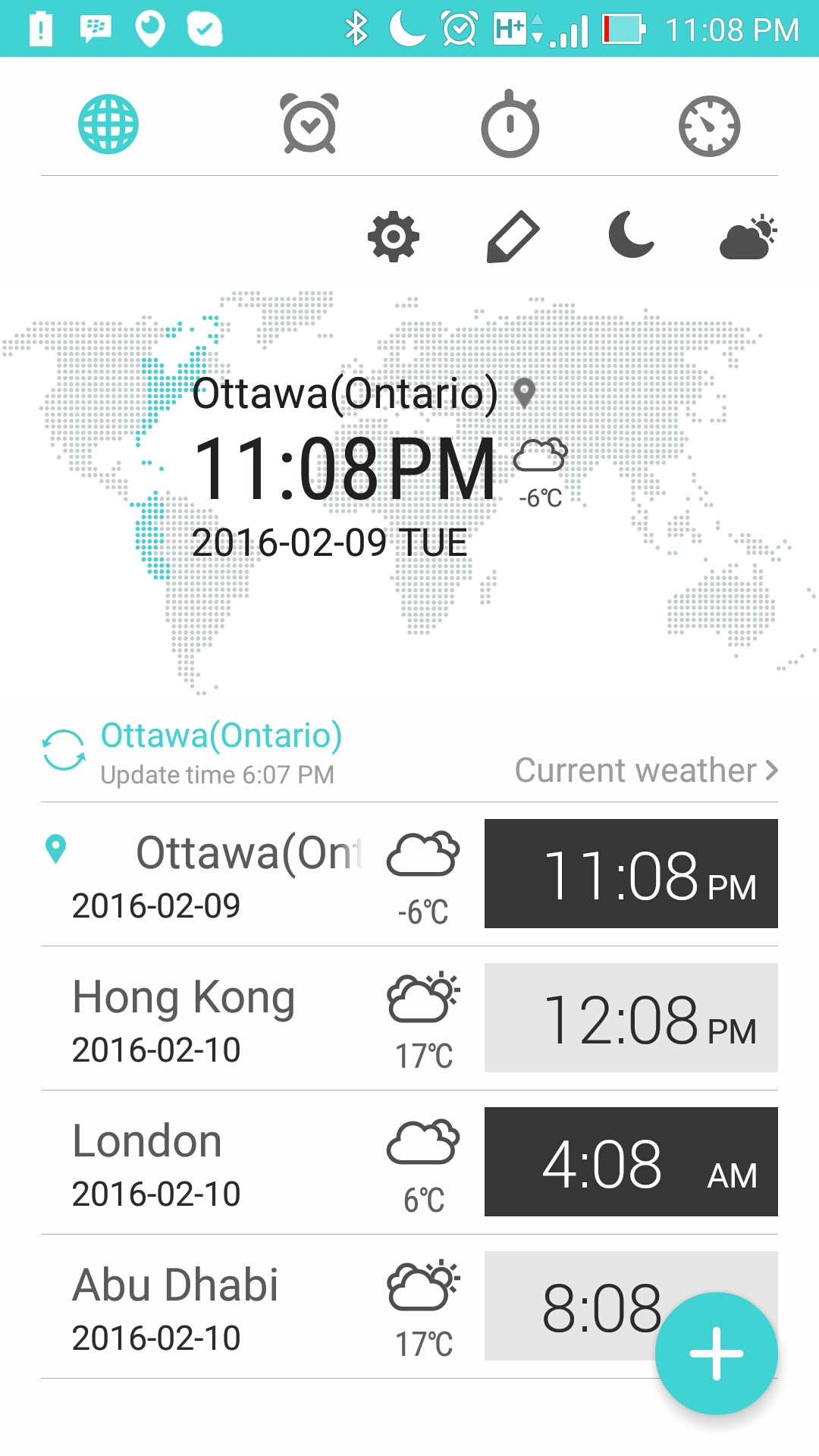**Descriptive Caption for Image:**

The image appears to be a screenshot from a mobile phone, featuring a variety of informational icons and details. At the very top of the screen is a thin aqua blue bar, populated with several icons. On the far left, there is a battery icon with an exclamation point next to a quote bubble, a location icon, and a cloud icon with a check mark. Moving to the right, there is a Bluetooth icon, a moon icon, and an alarm icon, followed by a white box labeled "H+." Further right, there is a signal bar icon, a horizontal battery icon with a red line indicating low charge, and on the far right, the time is displayed as 11:08 PM.

Below this top bar, there are four primary icons: a blue circle with overlapping ovals, a gray alarm icon, a gray stopwatch icon, and a clock icon. Beneath this row, a thin light gray line separates these icons from another set, which includes a gear icon, a pencil icon angled towards the bottom left, a dark gray moon icon, and a dark gray cloud icon with a sun peeking out from the upper right.

The background of the main screen prominently features a pixelated world map with the Eastern Time Zone highlighted in aqua blue, contrasting against the gray pixels representing the rest of the world. Below this map, the location "Ottawa (Ontario)" is displayed with the current local time of 11:08 PM and a cloud icon indicating the weather. The temperature is shown as -6°C. Directly beneath this information, the date "2006-02-09, Tuesday" is listed.

A section with additional time zones is positioned further down, featuring four locations: Ottawa showing 11:08 PM, Hong Kong at 12:08 PM, London at 4:08 AM, and Abu Dhabi at 8:08 AM. In the bottom right corner of the screen, there is an aqua blue circle with a white plus sign.